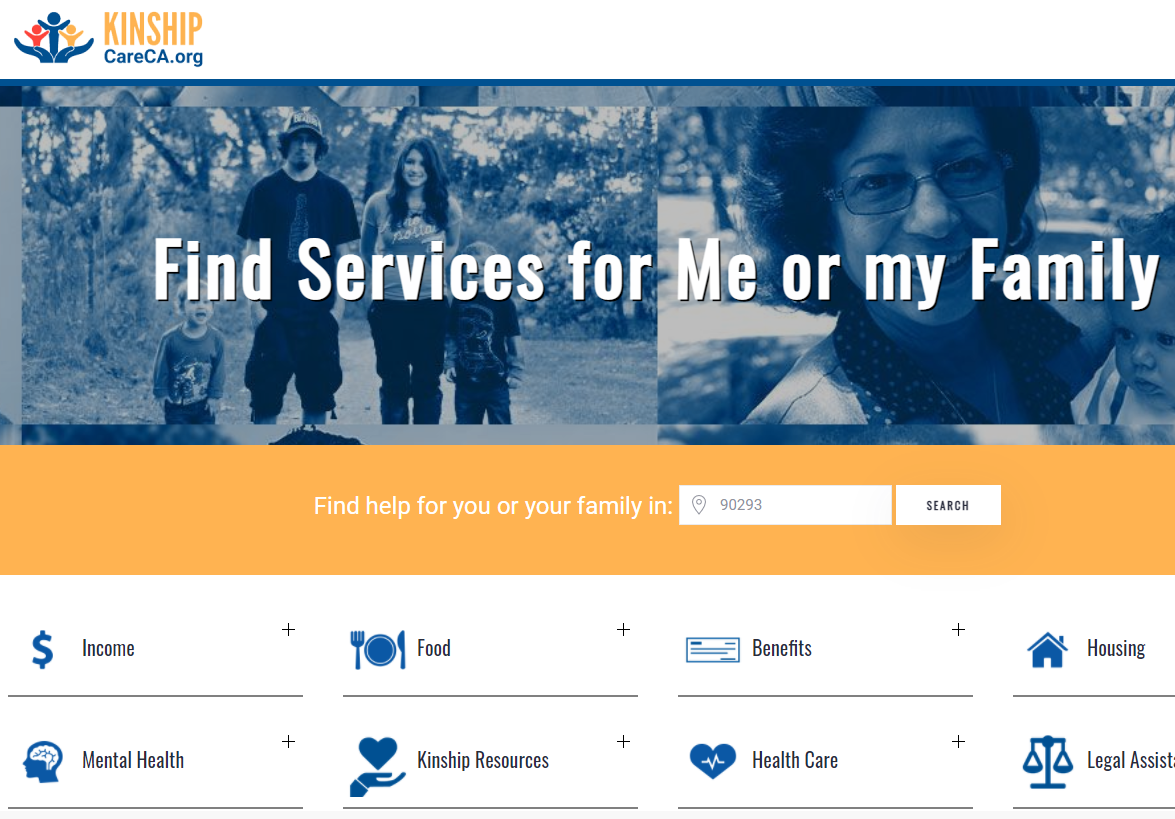The image is divided into several sections, each providing specific information and visual elements related to services and resources for families.

At the top left corner, a white section features a logo consisting of two blue shapes, possibly hands or leaves, accompanied by a trio of figures: one red, one blue, and one resembling an Amish person. Below this logo, the text "kinship" is prominently displayed, with "careca.org" written in blue underneath it.

The background transitions into a blue outdoor scene, where a family—a man, a woman, and two children—are visible. In an open white space within this background, the text "Find services for me and my family" is inscribed. Adjacent to this, on the right side, an older woman, possibly a grandmother, is shown holding a baby. This side is bordered by an Amish-themed design and includes the text "Find help for you and your family" in white font.

Below, there is a white search box with the placeholder text "09293" in gray. Adjacent to this, another box contains the word "Search" in black.

The lower part of the image features two rows of icons and tabs, each associated with different categories of services. Starting from the left in the first row, there is a teal dollar sign labeled "Income," a teal plate with a fork and knife labeled "Food," the word "Benefits" in black, and a teal house labeled "Housing." Each of these icons has a plus sign in the upper right-hand corner.

In the second row, from left to right, there is a blue icon of a brain inside a head labeled "Mental Health," an icon of a hand holding a heart labeled "Kinship Resources," an icon of a heart labeled "Healthcare," and a scale labeled "Legal Assistance." Each of these also includes a plus sign in the upper right-hand corner.

This detailed layout provides an organized and comprehensive overview of available services and resources tailored for families.